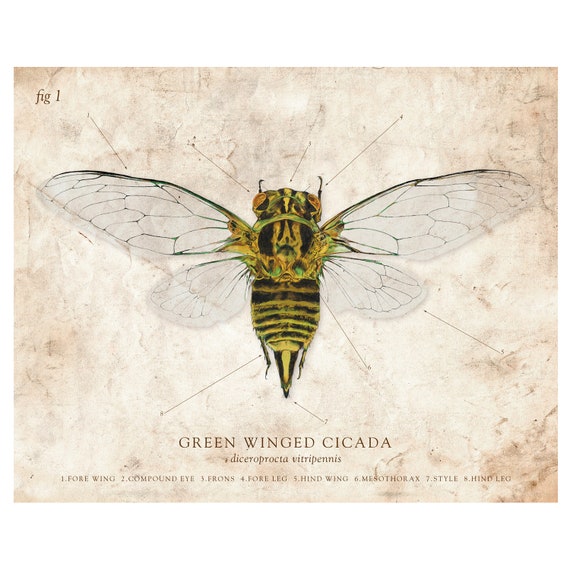The illustration depicts a green-winged cicada, identified at the bottom as "Green-winged Cicada (Diceroprocta vitripennis)." The image, labeled "FIG 1" in the top left corner, stands out on a backdrop designed to look weathered or marbled. The insect, viewed from above, combines features reminiscent of both a bee and a butterfly. Its body is primarily yellow with black stripes, and it has four wings: two larger transparent, gray-tinted forewings with fragmented shapes and subtle green coloration, and two smaller hindwings. The cicada has prominent yellow compound eyes, a pointed stinger, and antennae extending from its head. Below the cicada, a diagram labels various parts, including the forewing, compound eye, fronds, foreleg, hindwing, mesothorax, stile, and hind leg, each indicated with arrows pointing to their respective locations on the insect.